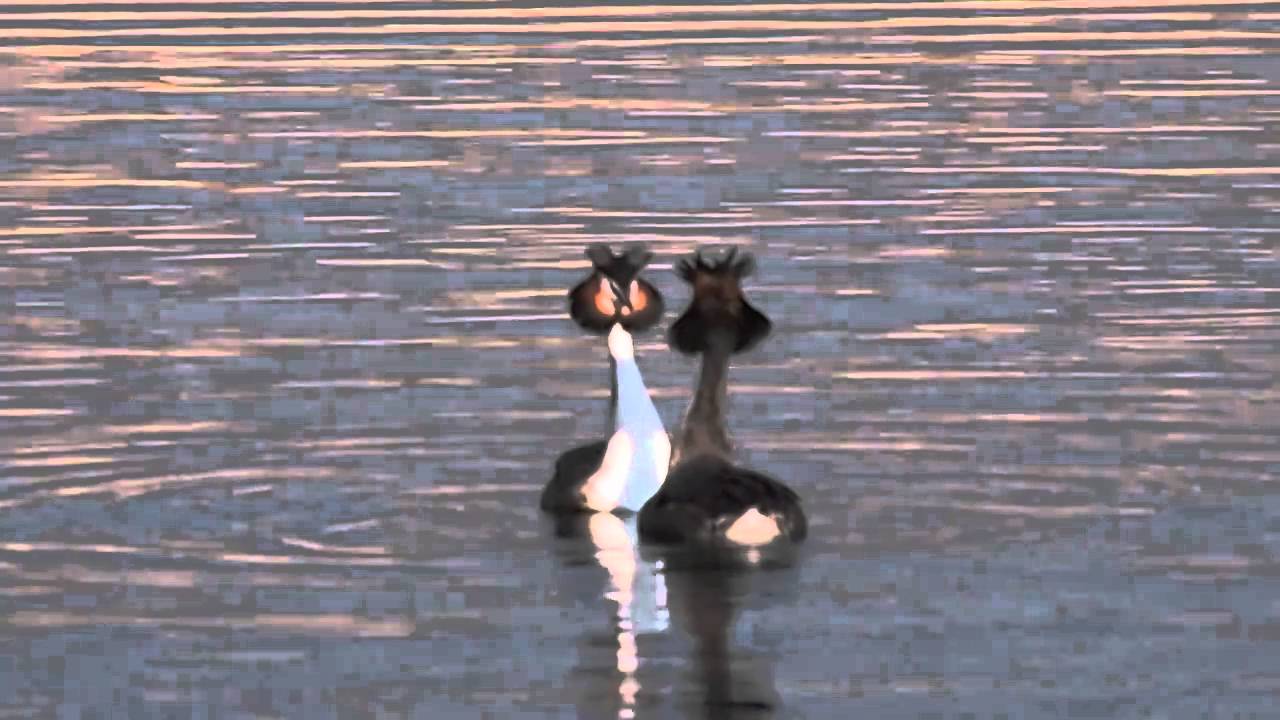This color photograph, though heavily pixelated and out of focus, seemingly captures a serene scene of two birds on a calm body of water, possibly a lake. The water presents a mix of blue with light reflections and hints of gray and pink, likely from a setting or rising sun, adding a harmonious and tranquil touch. The photograph's low resolution suggests it might be a still from a video or an image captured with a digital zoom, adding to its abstract, almost painting-like quality. In the center, two birds are visible, each mirroring the other. One bird is seen from behind, displaying an entirely black body except for a lighter spot on its tail. The other bird faces the viewer, its white and light blue neck and belly glowing against the water, while its eyes emanate a striking red. Both birds share a unique bulbous, onion-shaped head. Their reflections can be faintly seen on the calm surface, contributing to the overall ethereal and dreamy atmosphere of the image.